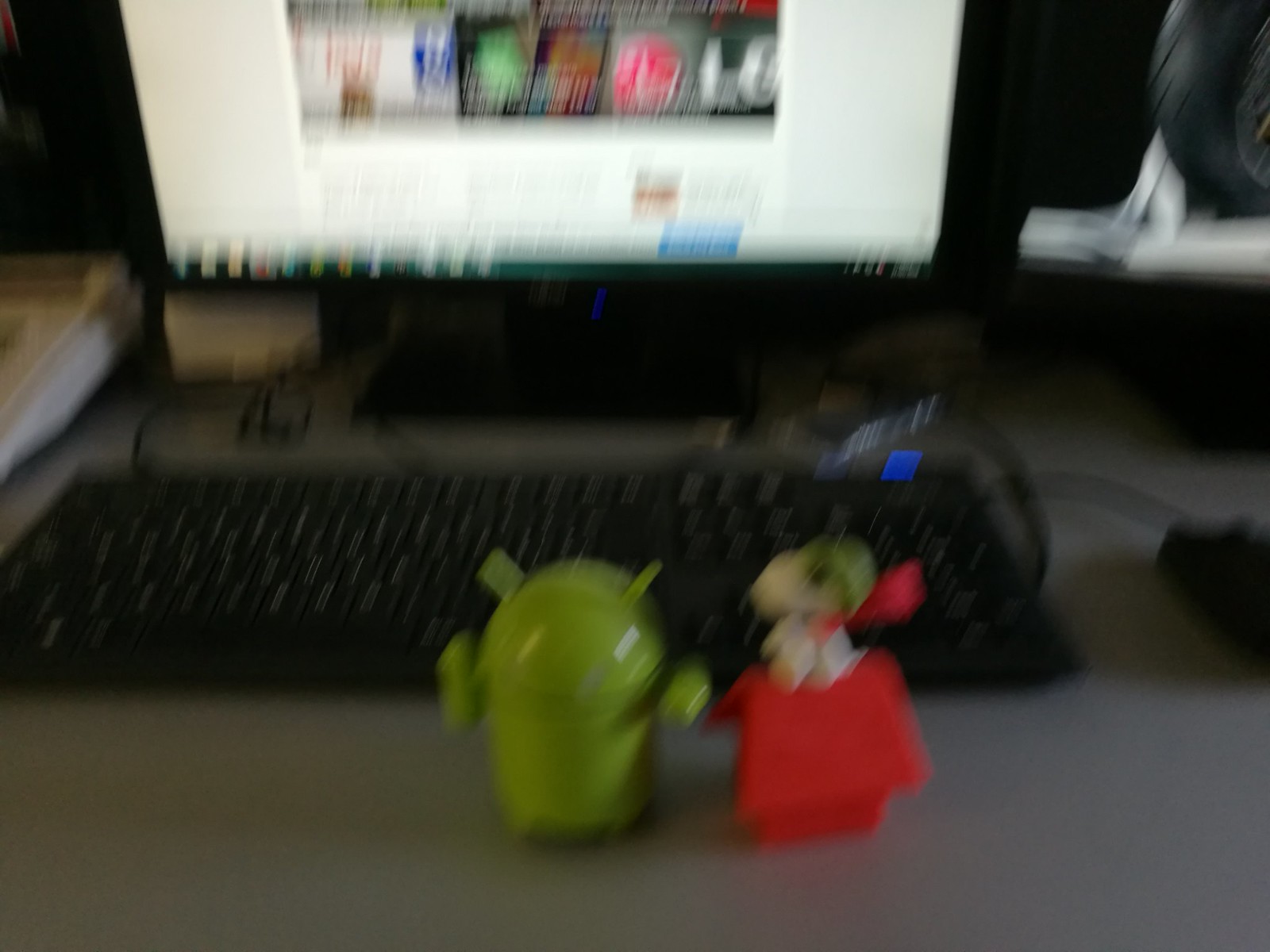This extremely blurry photograph captures a desktop computer setup, including a monitor with a black bezel, a corded keyboard, and a corded mouse placed on a gray table. The display screen shows an image bordered in white. In front of the computer setup, there are two notable models: one green cylindrical object that resembles a small robot from Star Wars, and a detailed figurine of Snoopy from the Charlie Brown series. Snoopy is depicted wearing a scarf and helmet, seated atop his iconic red doghouse. Despite the blurriness caused by a bumped camera, the elements and their arrangements within the photo are discernible.